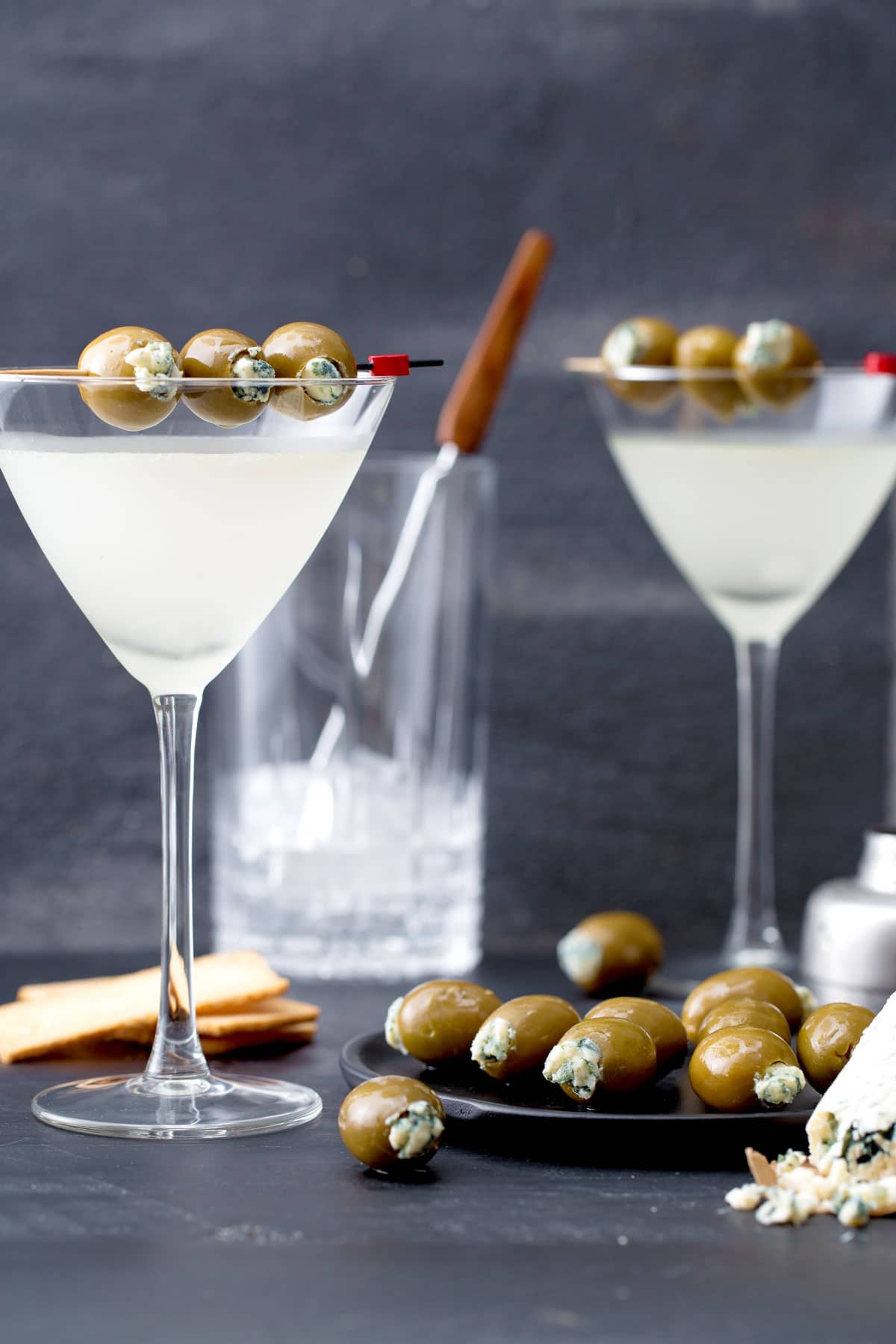The photograph captures a close-up scene with a gray background and gray table, featuring two martini glasses filled with a murky white cocktail, presumably martinis. Each martini glass is garnished with a skewer of three blue cheese-stuffed olives, with red-tipped ends, balanced across the top. Behind the leftmost glass, three thin crackers are positioned on the table. To the right of the rightmost glass, there's a black platter with around a dozen blue cheese-stuffed olives, with one olive having rolled off onto the table. An edge of a wedge of blue cheese is visible in the forefront to the right. In the background, there's a narrow, clear ice bucket with tongs with a wooden handle. Overall, the image is mostly gauzy and blurred except for the plate of olives and the leftmost martini glass, giving it a focused, yet stylishly soft, promotional feel. This entire setup is placed on what appears to be a black countertop, possibly made of stone like marble or granite.